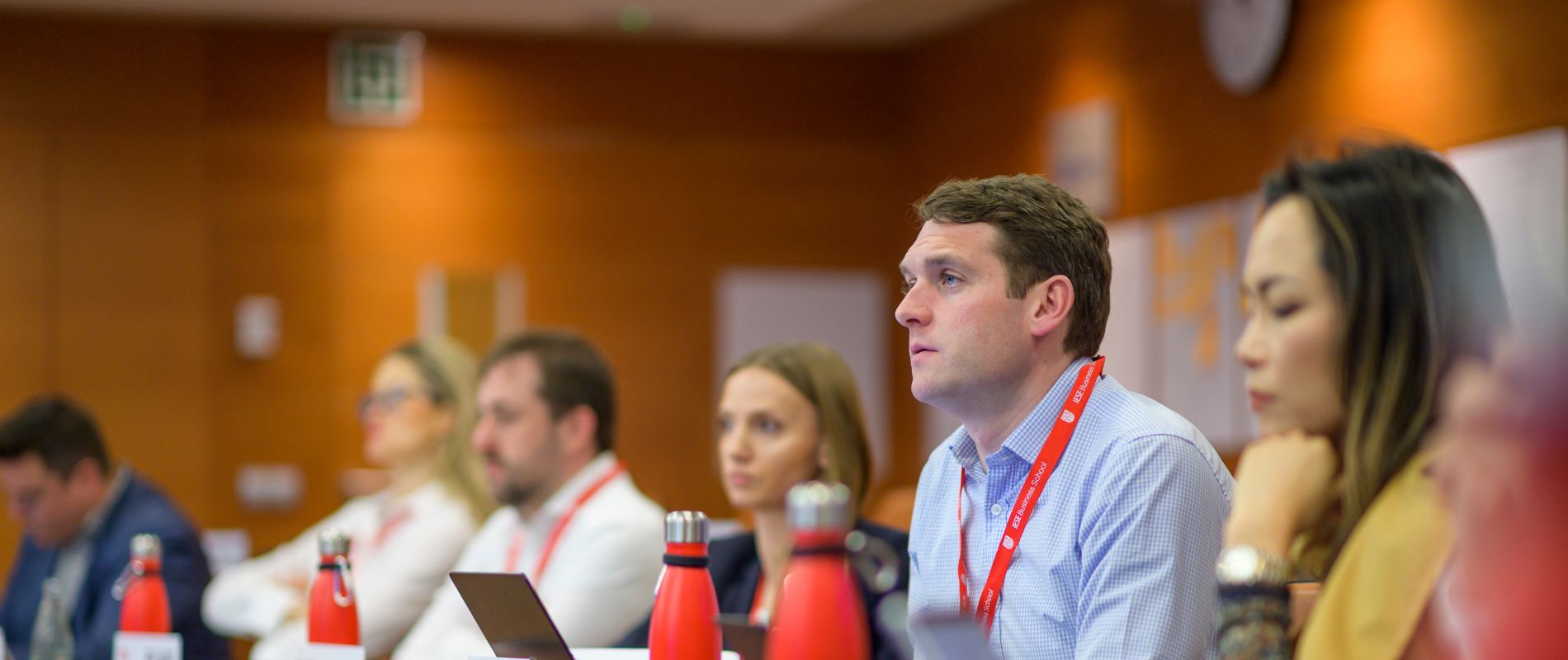The photograph depicts a group of six individuals seated in a row, likely at a conference or professional event, all appearing to be engaged in watching or listening to something off-camera. The setting, resembling a courtroom or panel discussion environment, features wooden walls and gray rectangular soundproofing panels.

Closest to the camera on the right side, a slightly Asian woman with long brown hair is somewhat blurred; she has her chin resting on her hand and her eyes closed. Next to her, and the clearest in the photo, is a man in a blue shirt with a red lanyard, leaning forward and intently staring ahead. Also seated at the table are several red-capped metal bottles, possibly containing water.

Following the focal man, the next person is a woman with long brown hair, who becomes more blurred with distance. Further on, a man in a white shirt appears next to her, followed by a woman with blonde hair and glasses, arms folded across her chest. At the far end of the row, another man in a blue shirt is looking downward. The participants, displaying a mix of cultural backgrounds, are dressed in business attire, suggesting a formal and professional gathering.